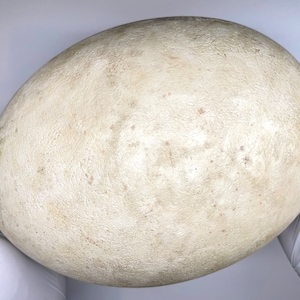The image depicts an object that is distinctly oval in shape, closely resembling either an egg or a polished stone. The surface of the oval object is an eggshell color adorned with small imperfections and light brown freckles, giving it an organic, slightly pitted appearance. The object is held between the fingers of a gloved hand, which are cropped within the photograph, adding a sense of scale. The background is a light lavender or gray tone, creating a neutral backdrop that highlights the object. The object seems to be nestled in a soft, cushioned surface, which appears white, hinting at a careful and delicate presentation. The photograph is small and square, about an inch and a half in height and width, suggesting an intimate and close-up view of the object, which could be perceived as either a large egg or an artfully shaped stone. The image captures the object's delicate texture and intricate details, making it a compelling subject of focus against the subdued background.